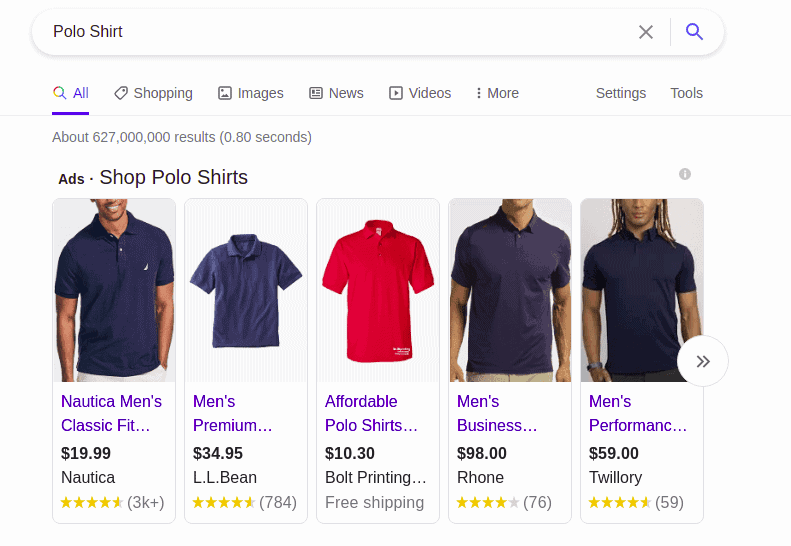The image displays a computer screen showcasing a search query for polo shirts. The search results include five advertisements prominently labeled "Shop Polo Shirts." 

1. The first result features a dark blue polo shirt from Nautica, specifically the Men's Classic Fit model, priced at $19.99. This item has received a five-star rating based on over 3,000 reviews.
   
2. The second polo shirt is also dark blue, labeled as a Men's Premium Polo from L.L. Bean. This shirt costs $34.95 and boasts a five-star rating with 784 reviews.

3. The third option is a red polo shirt marketed under "Affordable Polo Shirts" by Bolt Printing, priced at just $10.30 with the added benefit of free shipping.

4. The fourth image highlights a men's business polo shirt from Roan, priced at $98. This item holds a four-star rating from 76 reviews.

5. The final result is a Men's Performance Polo by Twillery, priced at $59. This shirt has garnered a perfect five-star rating from 59 reviews.

At the top of the search results, it is indicated that there are approximately 627 million results for this query. Below the search options, there are additional tabs for "All," "Shopping," "Images," "News," "Videos," and "More."